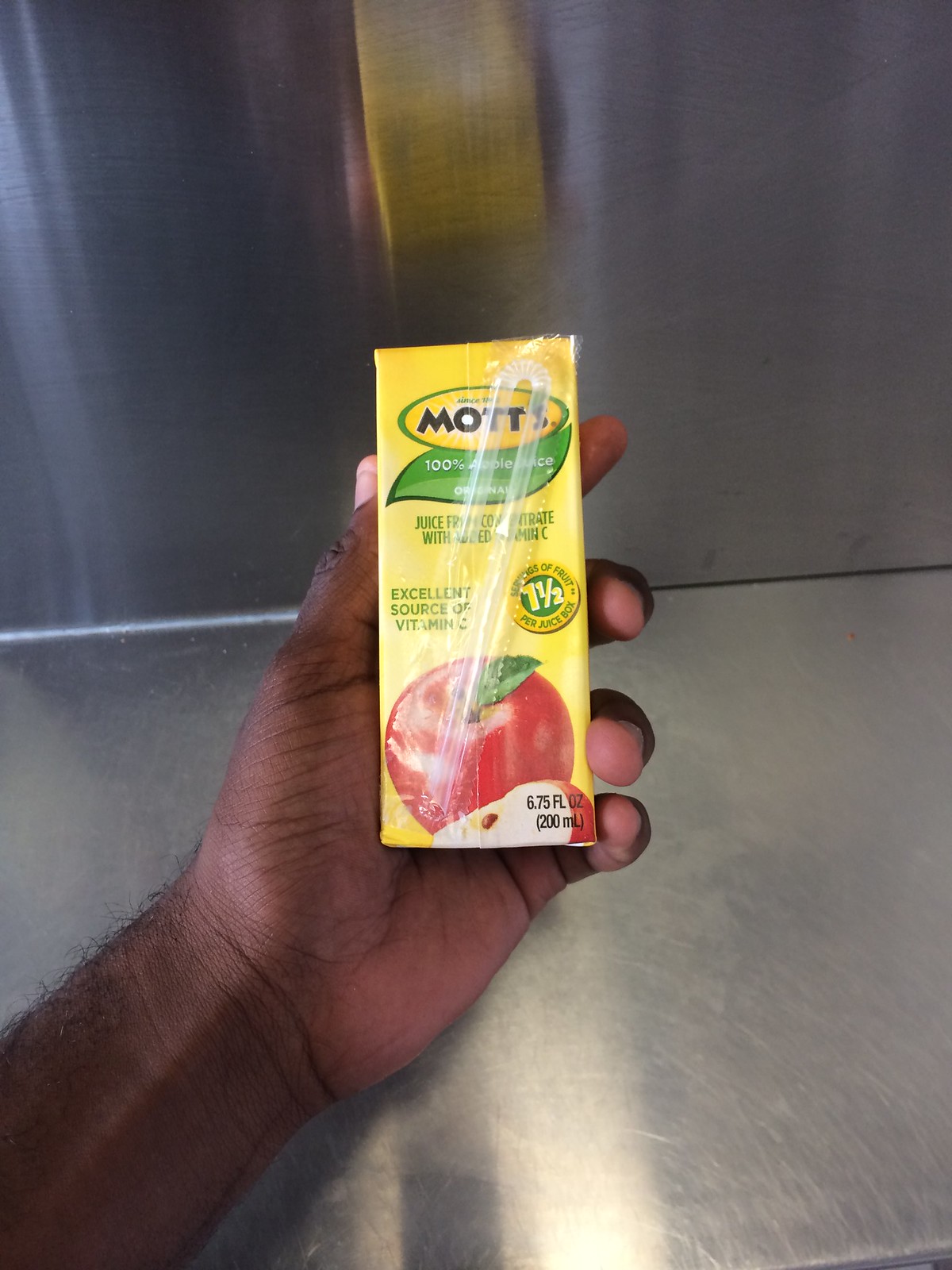This is a close-up photograph of a man's left hand, noticeably hairy, holding a small single-serving Mott's apple juice carton. The yellow carton features a red apple with a green leaf and a slice of apple. The front of the carton has a little attached straw. Text on the carton includes "100% apple juice," "original," "juice from concentrate," and "excellent source of vitamin C," alongside additional nutritional information. The hand is resting on or near a chrome or metallic surface, with reflections of the juice box visible at the top of the image and a metal wall or object in the background. The juice box contains 6.75 fluid ounces of apple juice.